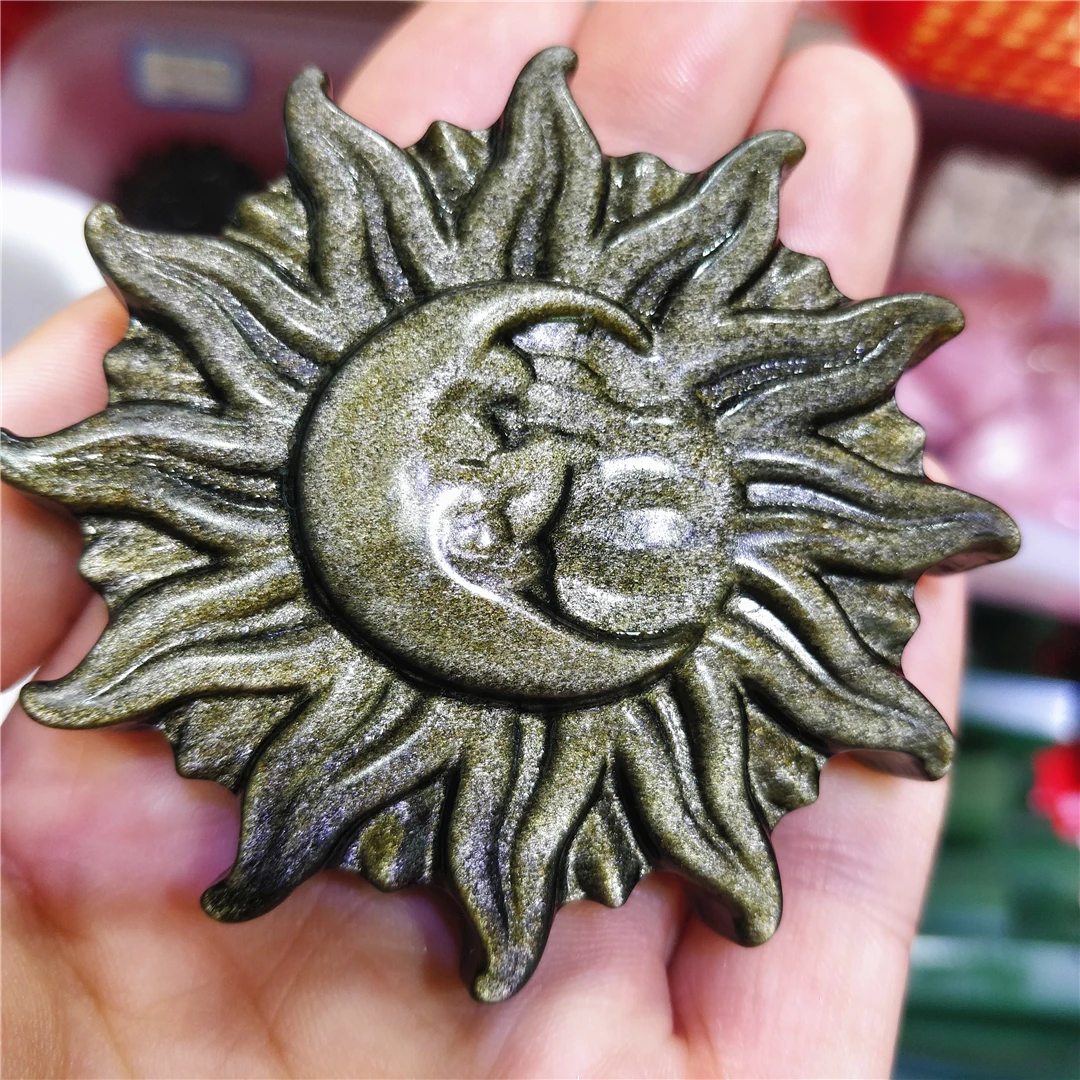The image depicts a close-up view of a Caucasian hand, palm up and open, holding a unique art piece made of what appears to be metal with a brownish-golden patina, resembling bronze. The object, which nearly spans the width of the hand from the first knuckle to the center of the palm, is shaped like a sun or a flower with curved rays featuring lines in their centers and a scalloped edge. At its core, the object contains a central circle with a carved crescent moon and additional curved lines within the moon. The metallic surface shines as it catches the light, reflecting a glossy sheen. The background is blurred with hues of pink and green, slightly visible but out of focus, drawing attention to the detailed engravings and textures of the sun-moon object in the hand. The intricate engravings and the overall sun-like appearance, including the rough, bumpy texture of the moon, add to the richness of the visual detail.